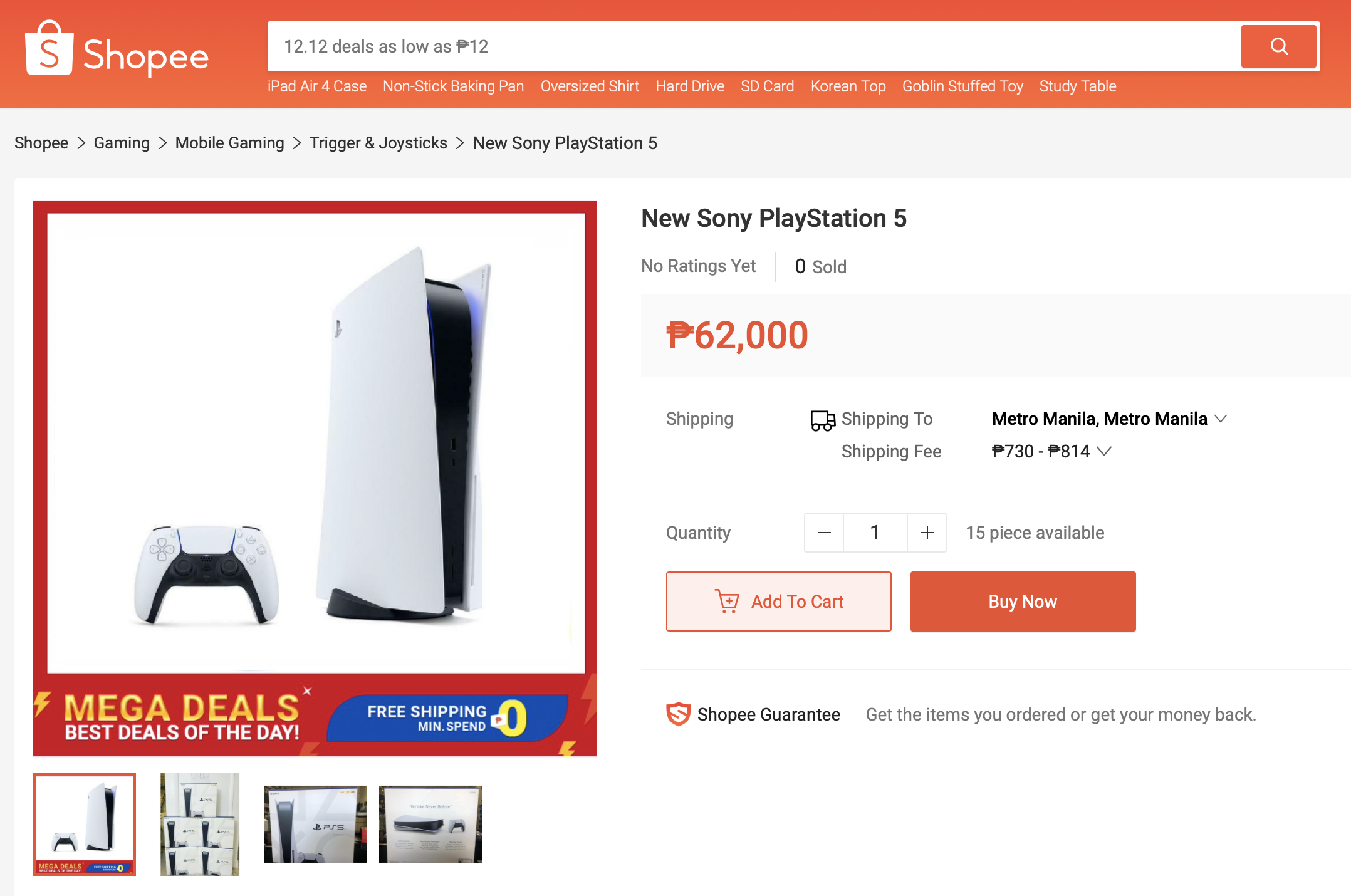The web page features a prominently placed, vibrant orange-red rectangle at the top of the page. Inside this rectangle is a contrasting white rectangular section with a logo featuring a shopping bag with an "S" on it, accompanied by the brand name "Shopee." The text in the white rectangle promotes "1212 deals as low as 12" and includes a search icon. Adjacent to this are categories listed as "shopping," "gaming," "mobile gaming," "trigger and joysticks," and "new Sony Playstation 5".

On the left side of the web page, there is a large red rectangle displaying a PlayStation 5 console and controller, both colored in sleek white and black. The section advertises "Mega Deals," "Best Deals of the Day," and features a "Free Shipping" banner in yellow and white, with "free shipping" highlighted additionally in blue.

To the right of the PlayStation 5 image, the product is described with the text "New Sony Playstation 5" followed by "no rating yet." The price is listed as "P62,000" with shipping available to Metro Manila. The stock information indicates "15 pieces available," with the default quantity set to "1".

At the bottom, there is a red square with a white interior featuring a shopping cart icon and the text "Add to Cart". Beside it, a solid red rectangle with "Buy Now" written in white provides a clear call to action.